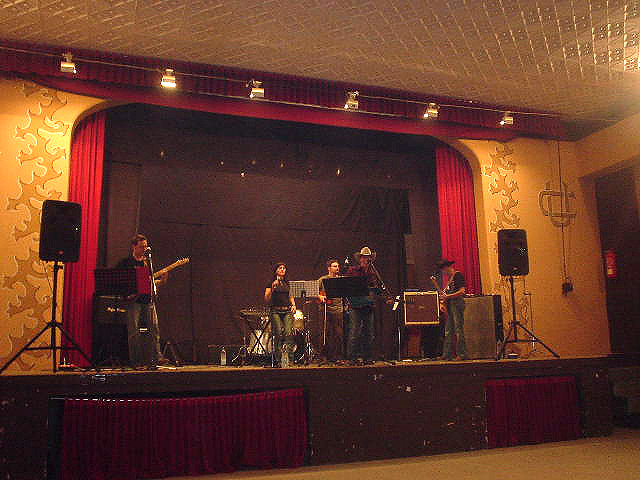In the photograph, a band is energetically performing on an elevated stage with a front facade painted brown, revealing white scrapes underneath. The stage front is adorned with small maroon curtains, while the backdrop features similar red curtains set against a yellow wall with a gold, thorny pattern on either side. The central figure, a man in a black t-shirt, blue jeans, and a cowboy hat, is playing an electric guitar and singing into a microphone positioned close to his face. To his right, a woman in blue jeans and a black short-sleeved t-shirt passionately sings into a microphone. Another man to the left of the central figure, potentially holding a fiddle bow, and another guitarist or bass player on the far left complete the lineup. The atmosphere is further enhanced by bright yellow lights shining down from the ceiling, illuminating the band during their performance. The audience remains unseen, adding a sense of mystery to the lively scene on stage.